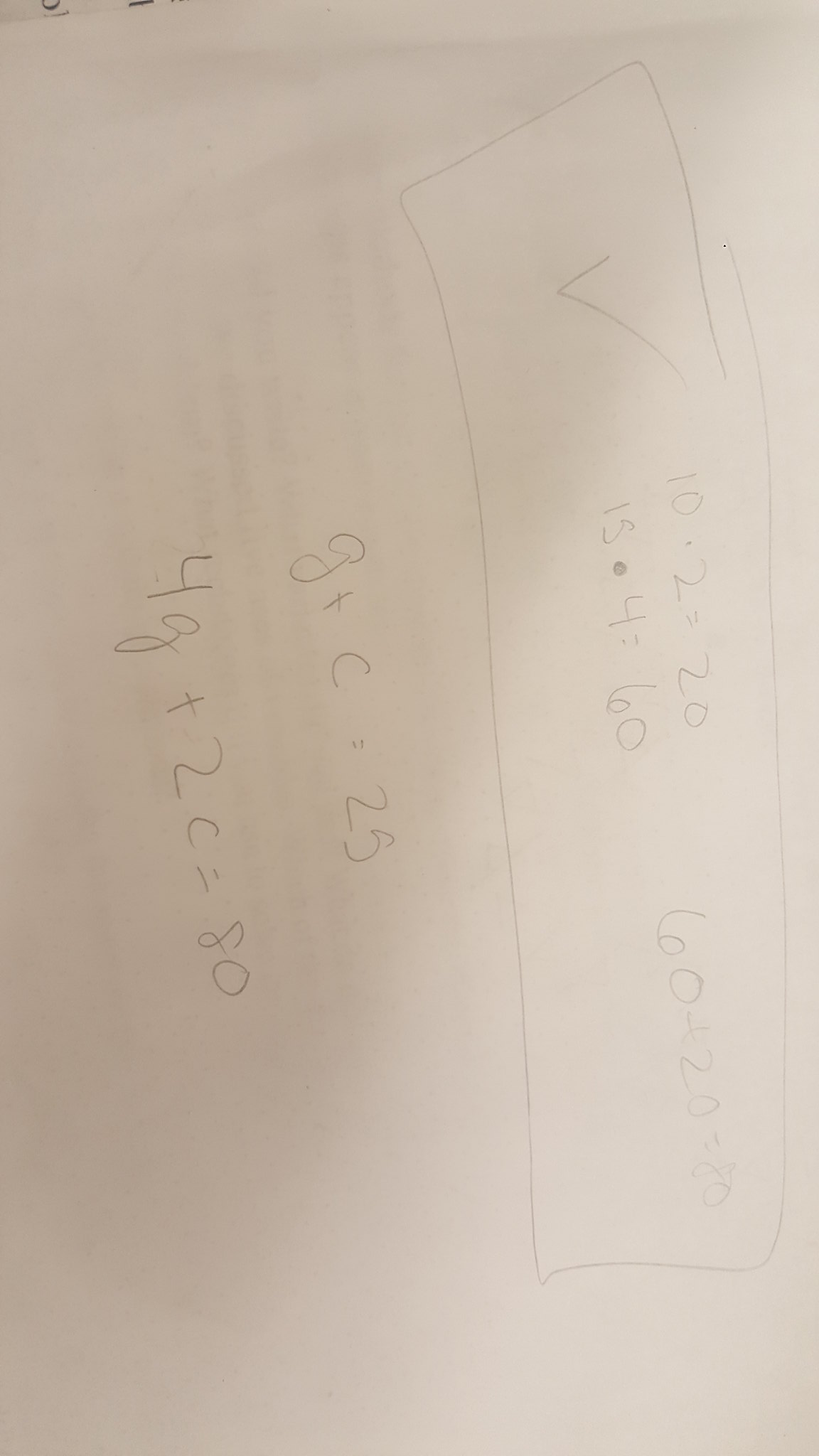In the photograph, a disoriented sheet of paper lies atop an open textbook, displaying a series of algebraic calculations recorded in pencil. To properly read the content, one must tilt their head to the side since the paper is placed in an unconventional, sideways orientation. Among the notations:

- A square at the top highlights the straightforward product calculations: \(10 \times 2 = 20\) and \(15 \times 4 = 60\), summing up to \(60 + 20 = 80\).
- Below, equations involving variables G and C are noted: \(G + C = 2G\) and \(4G + 2C = 80\), suggesting a problem where G and C might represent specific values.
- The writing appears crisp against what seems to be white paper, although a subtle filter effect is present, possibly due to ambient lighting or a digital overlay.

Additional marks, such as a check mark adjacent to the initial formulas, hint at verified steps in the problem-solving sequence. Despite the detailed mathematical entries, the specific meanings of G and C remain unidentified, leaving their context ambiguous. A faint overlay of the textbook's text serves as the backdrop, subtly reinforcing the academic setting of the scene, though the exact environment remains unstated.